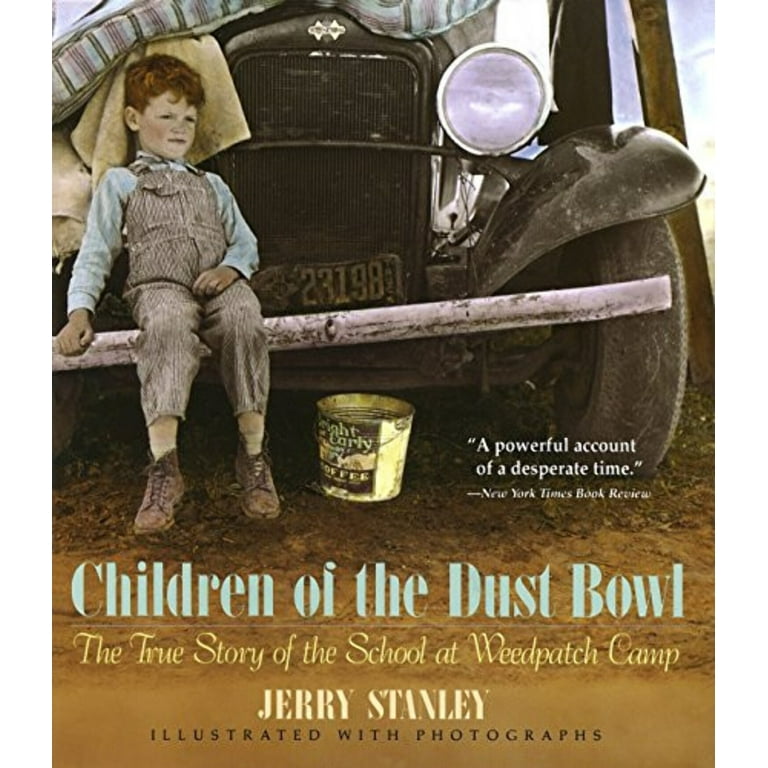The poster is a vintage scan for a book titled "Children of the Dust Bowl: The True Story of the School at Weed Patch Camp" by Jerry Stanley, illustrated with photographs. It features a powerful recommendation from the New York Times Book Review, stating, "A powerful account of a desperate time." The sepia-toned photograph on the poster depicts a small Caucasian boy with short, reddish-brown hair, dressed in 19th-century attire. He wears overalls with suspenders, a light blue shirt, stockings, and brown lace-up boots. The boy is seated on the bumper of an old automobile, which appears to have a mattress and blanket tied to its roof. The car is parked on a barren, dirt-covered ground. A license plate on the car reads "23198," enhancing the sense of authenticity and historical context. The title and text are positioned near the bottom edge of the image, beneath the car, in bold black font.